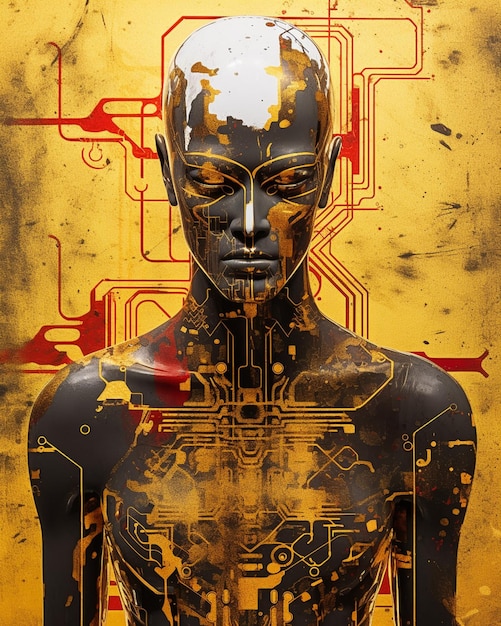The image depicts a highly detailed piece of futuristic artwork likely created using computer graphics. The central figure is a dark gray, almost black humanoid, reminiscent of a mannequin or robot, with intricate techno-like yellow lines and circuitry patterns adorning its body. This figure exudes a technological aesthetic akin to characters from sci-fi movies like "The Matrix." 

The background predominantly features a striking yellow color with red lines intertwined, suggesting a network of computer circuits or wiring. Additional red splotches appear on the figure's left shoulder, enhancing its industrial and worn look. The head of the figure is notably white with apparent signs of decay or damage, adding to the futuristic and distressed appearance. The overall composition juxtaposes the sleek, modern lines of technology with elements that suggest wear and deterioration, creating a compelling cybernetic visual narrative.